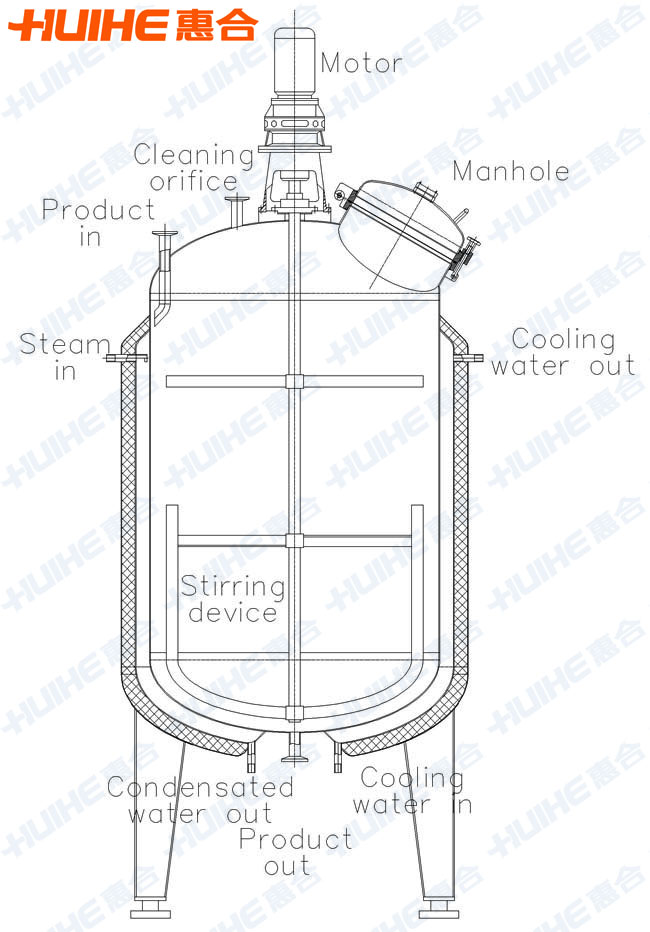This black and white schematic drawing represents a detailed diagram of a water storage or processing device. Prominently, H-U-I-H-E is inscribed in orange at the top right corner, accompanied by Japanese characters, with a watermark of this text repeated diagonally across the image.

At the top of the drawing, the motor is situated in a small box, which connects to a larger cylindrical component via a neck segment. This cylinder is approximately three inches long and one inch wide. Internally, the cylinder is delineated with various diagrams: one runs vertically through the center, and four others run horizontally.

In the top right section of this main structure, the manhole is indicated next to a small jug-like figure. Below this, the term "cooling water" is labeled in black. Supporting structures include two legs under the main cylinder, labeled as either steel or metal. Several specific ports and lines are marked on the image: 

- Left side features:
  - "Steam in" near the top.
  - Two additional small raised pieces labeled as "cleaning orifice" and "product in."

- Right side features:
  - "Cooling water in" near the front leg.
  - "Condensated water out" on the left near the front leg.
  - "Product out" at the bottom center near a valve.
  - Two hoses extend from the top and wrap around toward the bottom.

Additionally, there is a "stirring device" indicated midway down the diagram. This comprehensive illustration assists in understanding the operational and functional elements of the device.